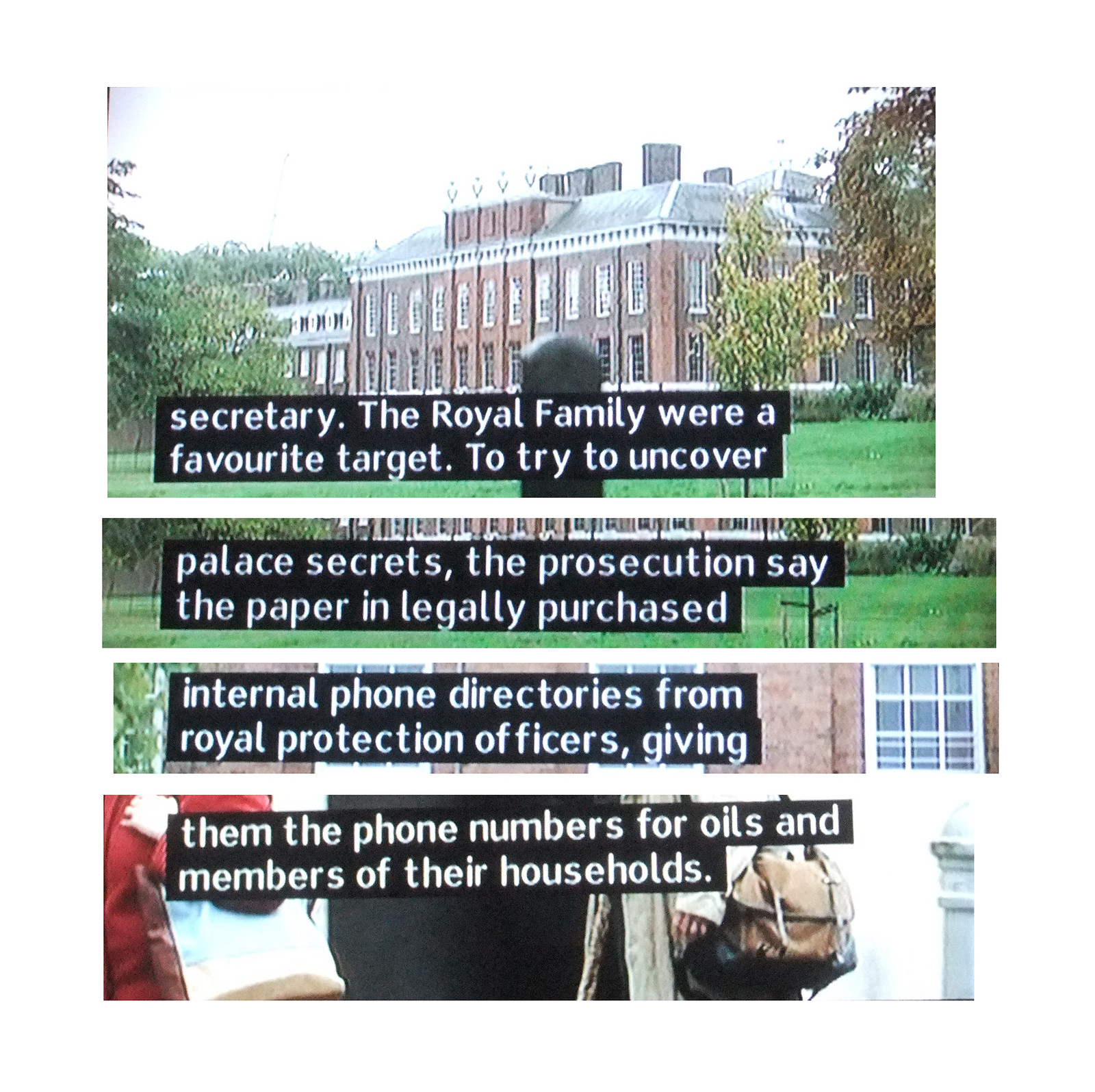The image consists of four distinct frames, taken from a television screen displaying a teleprompter. The text across the images appears to focus on revelations concerning the Royal Family, with a context that suggests it is from the UK, potentially London. 

1. The first image at the top has the caption: "The Royal Family were a favourite target, to try to uncover..."
2. The second image's text reads: "Palace Secrets, the prosecution say the paper is illegally purchased."
3. The third image displays: "Internal phone directories from Royal Protection Officers giving..."
4. The fourth and final image concludes with: "them phone numbers for VIPs and members of their households."

Together, the caption reads: "The Royal Family were a favourite target, to try to uncover Palace Secrets. The prosecution say the paper is illegally purchased, internal phone directories from Royal Protection Officers giving them phone numbers for VIPs and members of their households."

This series of images likely pertains to a legal case or investigation involving the unauthorized acquisition of sensitive information related to the Royal Family.